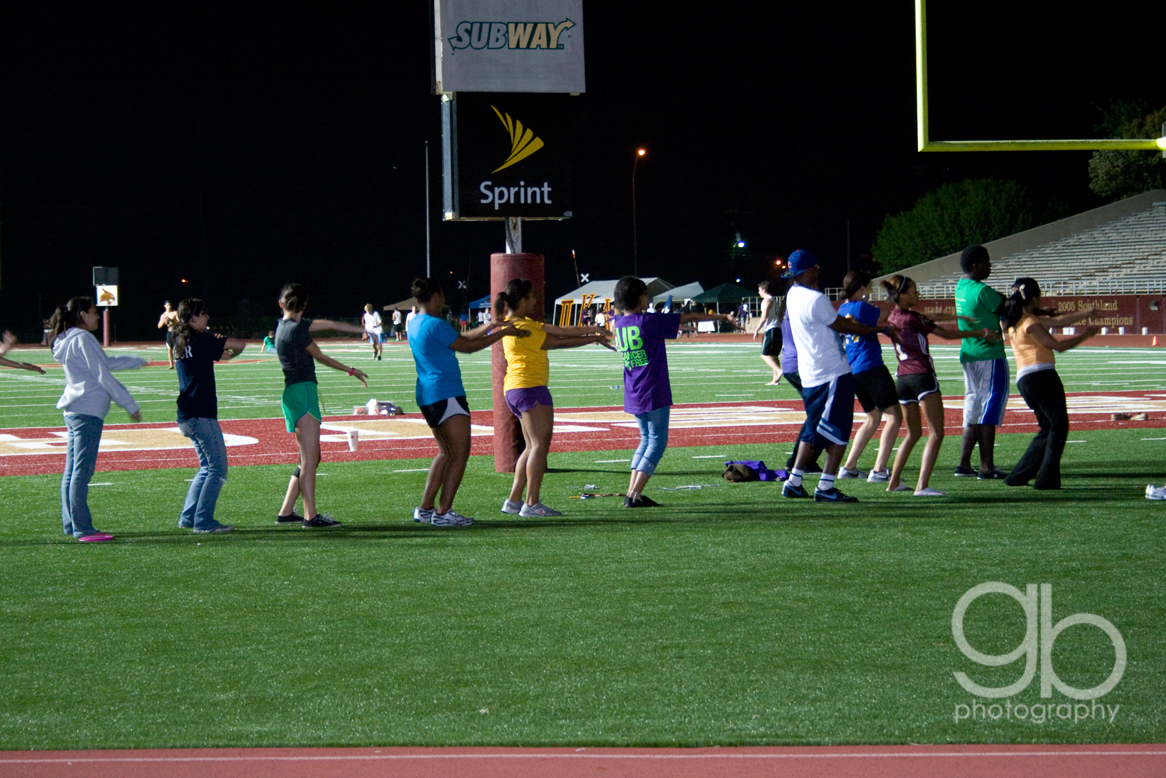The photo captures a nighttime scene in the end zone of a football stadium. The vividly-painted end zone features shades of red, gold, and white. A group of approximately ten people, mostly women but with a few men, are engaged in a synchronized line dance that resembles the Macarena. They are positioned on the green grass with their arms extended in front of them and legs slightly apart. Most participants are dressed in shorts, indicative of warm weather, while some opt for jeans. The prominent yellow goalpost stands out in the background, flanked by large, illuminated advertising signs for Sprint and Subway. The stadium stands appear empty, adding an eerie calm to the electric atmosphere on the field. A logo reading "GB photography" is visible in the bottom right corner of the image.